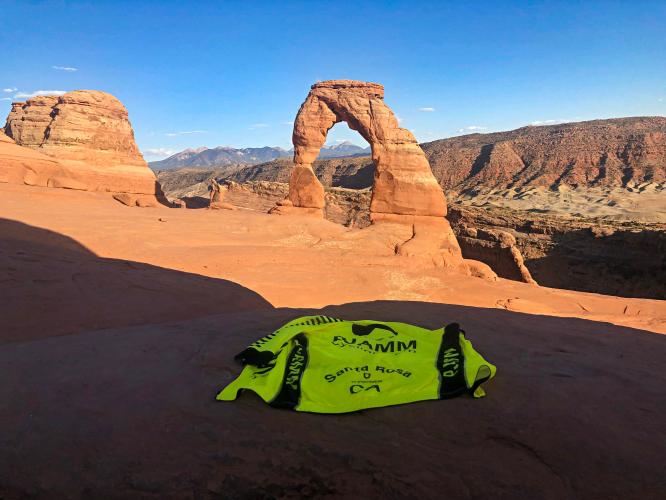This photo captures an expansive desert wilderness scene resembling the Plains region in Nevada or Arizona, possibly near the Grand Canyon. The central focus is a stunning rock formation featuring a natural arch, standing proudly above a deep canyon. To the left of this formation is another solid, orangish rock structure. In the background, massive mountains rise, their snow-capped peaks contrasting beautifully against a bright, almost cloudless blue sky. The photo is taken from a shaded area, highlighting the sunlit scene ahead. In the foreground, resting on the ground in the shadow, is a neon yellow and black jacket with some unidentified advertising imprint, possibly from Santa Rosa, California. This striking landscape, with its sandy hues and dramatic geological features, encapsulates the raw beauty of the desert.